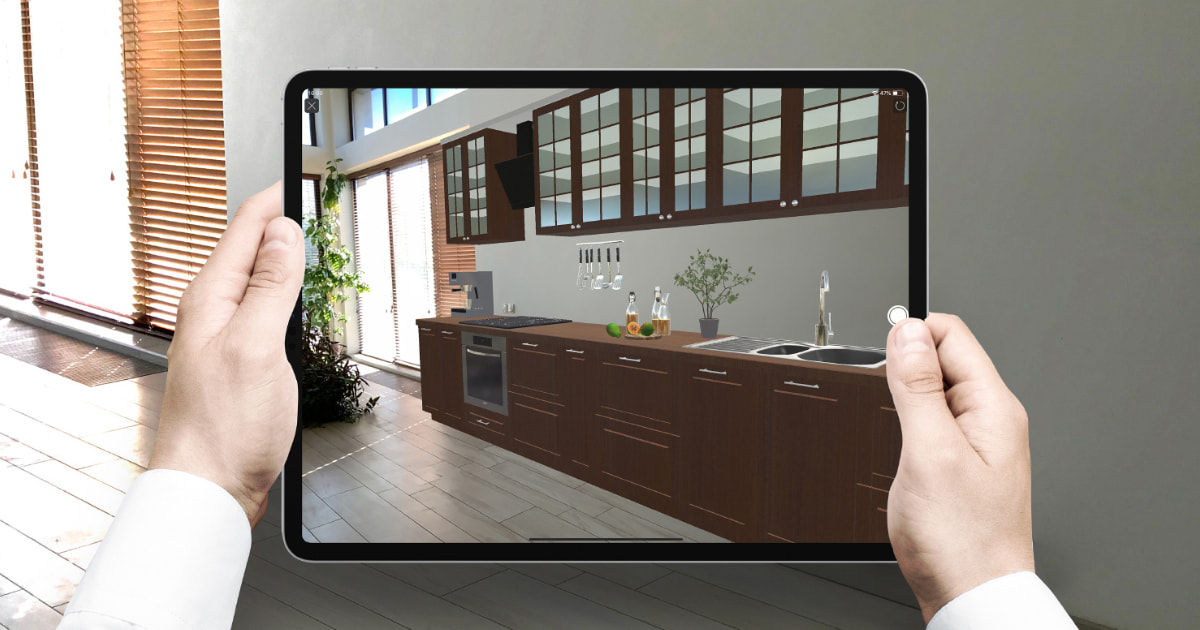In this detailed photo, a man, identifiable by his Caucasian hands and the white cuffs of his shirt, is holding an iPad that displays a carefully rendered 3D design of a kitchen. The image on the tablet showcases a modern kitchen with several notable features: brown cabinetry, an oven, a sink, and multiple overhead cabinets with glass panes. Utensils such as steel spoons hang from a wall rack, while a plant and some green produce, likely avocados, add a touch of nature to the scene. A coffee maker is also visible on the countertop. The kitchen scene depicted on the iPad includes a sliding door, suggesting access to another room or an outdoor space, with bright daylight streaming in. In the room where the man stands, visible behind the tablet, there is a gray wall and a window fitted with brown blinds, casting light onto a hardwood floor.